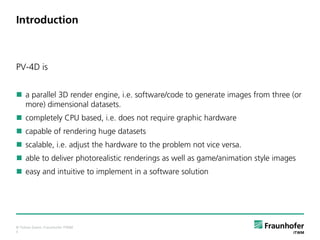This image features an introductory slide for a piece of computer software. At the top left corner, the word "Introduction" is prominently displayed in black letters against a completely white background. Directly below this title, the name of the software, "PV-4D," is presented. Underneath this, a series of detailed bullet points, each marked by green bullets, outline the software's features as follows:

- A parallel 3D render engine and IDE software/code designed to generate images from three or more dimensional datasets.
- Completely CPU-based; does not require graphic hardware.
- Capable of rendering huge datasets.
- Able to deliver photorealistic rendering as well as game animation-style images.
- Easy and intuitive to implement in a software solution.

Beneath the bullet points, a green line spans the entire width of the image from left to right. In the bottom left corner, there is a small segment of black text. On the bottom right, the company branding for Fraunhofer is visible, featuring a green emblem to the left of the word "Fraunhofer."